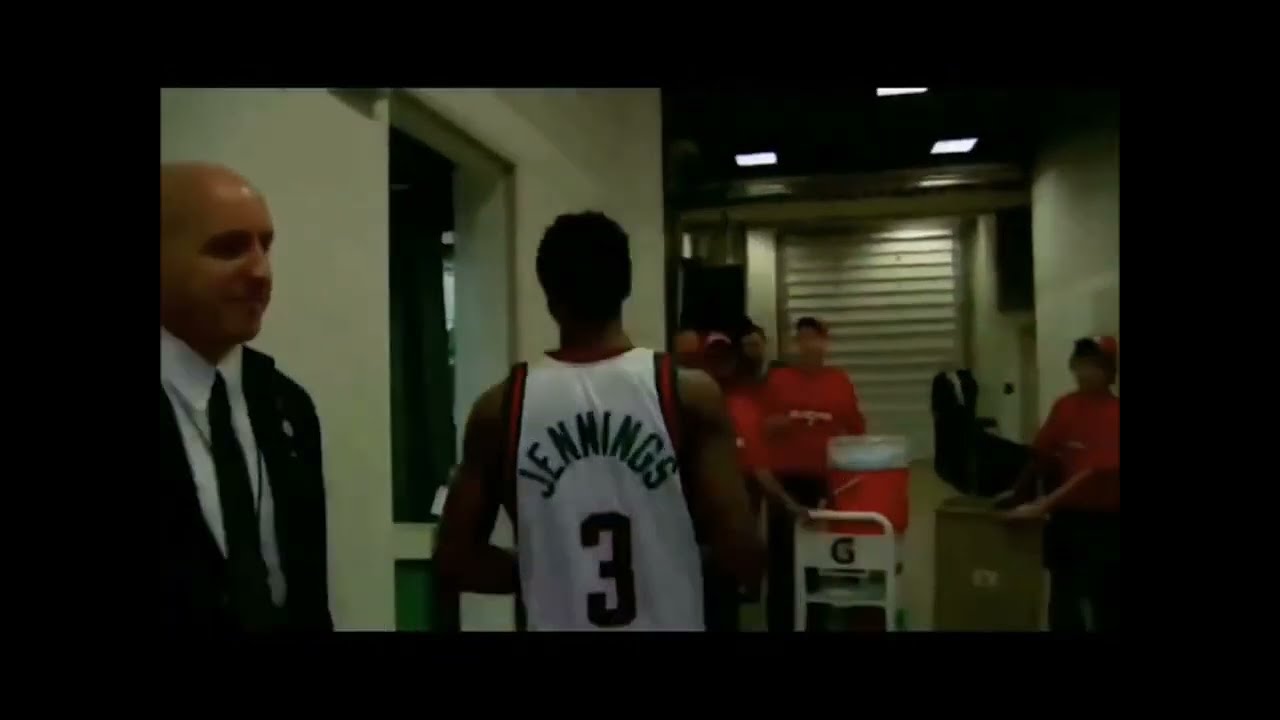In this blurred image of a fast-paced basketball game, two teams are vying for control of the court. One team, dressed in white jerseys with red text, are identified as the Chicago Bulls, while the opposing team is wearing green jerseys. A player in a green jersey appears to be executing a slam dunk towards the hoop, which features a white net and a glass backboard supported by a white arm. Above the hoop, a red LED shot clock and an orange timer display the remaining time in the quarter. The wooden court is surrounded by a busy, but blurry, crowd and a red advertisement for Budweiser with a white wavelike design lines the sidelines. This image, despite its lack of clarity, captures the intensity and excitement of a moment in what may be an important, possibly historic basketball game.